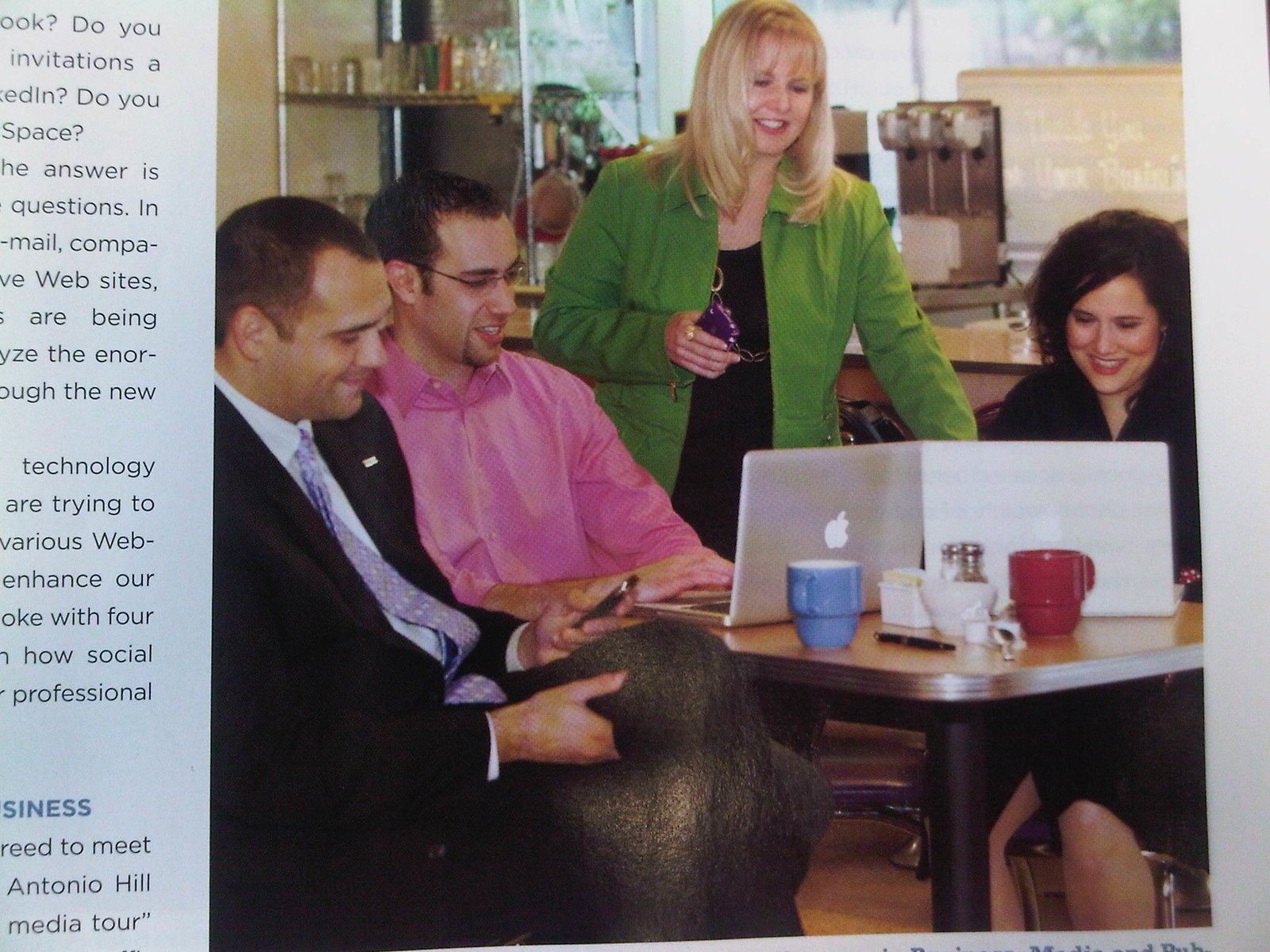The vibrant image, seemingly from a magazine, depicts a lively scene at a small, square wooden table with a single pole for support, surrounded by a textured yellow wall. Seated around the table are four individuals engaged in what appears to be a collaborative discussion. The table is adorned with two silver Apple MacBooks facing away from the camera, various coffee cups, a selection of packets of sugar, salt and pepper shakers with silver tops, and a black and silver pen.

From left to right: a man in a sharp black suit, accompanied by a white shirt and a distinctive blue tie, is engrossed in his phone, typing with his left hand. Adjacent to him, another man in a pink long-sleeve collared shirt and black-framed glasses is focused on his MacBook. Standing between them, a woman with blonde hair wearing a green jacket over a black dress is holding a phone with a purple case in her right hand. She appears to be gesturing or possibly showing something to the woman sitting next to her. This seated woman, sporting a black dress and long black hair, is also looking at her open MacBook, which seems to have a possible white glare.

The cheerful atmosphere is underscored by the smiles shared among the group. In the backdrop, a metal shelf stocked with various glasses—including a noticeable red and green one—and possibly an ice cream maker, suggests a restaurant setting. This image captures a moment of engaged interaction among the four, highlighting both their focus on technology and the cordial human interaction within a cozy cafe environment.